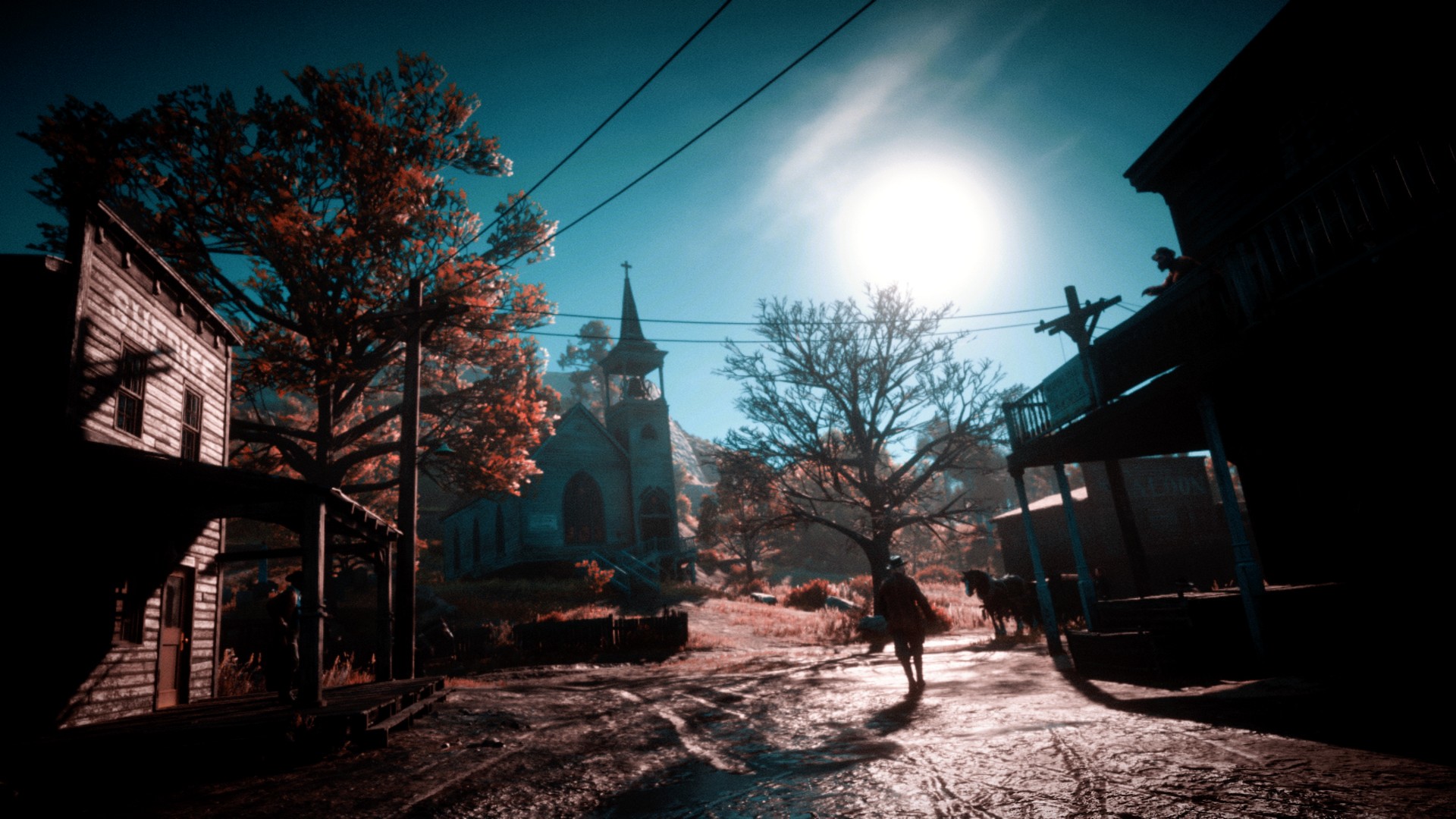In this rectangular photograph set against a vibrant blue sky, the scene unfolds reminiscent of a classic Western film. The foreground features a dirt road flanked by wooden buildings with low-lying porches, creating an authentic Old West ambiance. Off to the far distance, you can spot the silhouette of a church steeple, adding an air of bygone days to the image. Positioned to the lower right, a horse stands in front of a building, its form appearing as a stark silhouette against the brighter elements. A solitary figure, clad in a cowboy hat and wearing a cape that drapes over his attire, walks away from the camera, enhancing the nostalgic feel of the scene. Despite the historical look, the presence of two sets of telephone wires—one stretching diagonally from the lower left to the upper right, and another extending horizontally in front of the church steeple—blends modern elements into this otherwise timeless snapshot.